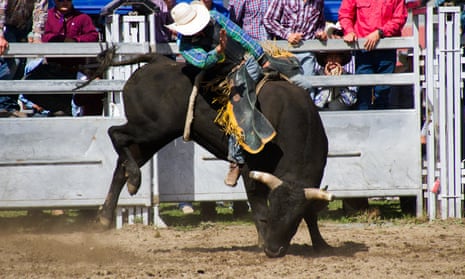This vibrant photograph, likely taken at a rodeo, captures an intense bull-riding moment in stunning detail. Central to the image is a black bull with white horns, vigorously bucking in an attempt to dislodge its rider. The bull's head is dipped towards the brown dirt of the arena, its mouth almost touching the ground, and one of its hind legs is lifted high, kicking up dirt behind it. The rider, clad in a blue plaid long-sleeve shirt and black chaps, is perched firmly on a black harness, his white cowboy hat tilted as he raises one hand in the air. His left hand holds the reins tightly, showcasing his determination to stay on the bull. 

In the background, there are metal barriers that separate the action from a crowd of spectators. These onlookers, many dressed in plaid, are partially obscured, with only their torsos visible due to the framing of the photo. A person in a red shirt and another in a checkered blue and white shirt stand out among the crowd, who watch the thrilling event unfold from behind the grayish fence. Behind the barriers, the ground transitions from the dirt-filled arena to patches of grass. The clarity of the photograph brings the chaotic energy of the rodeo to life, with dust particles visibly suspended in the air, emphasizing the bull's powerful movements.